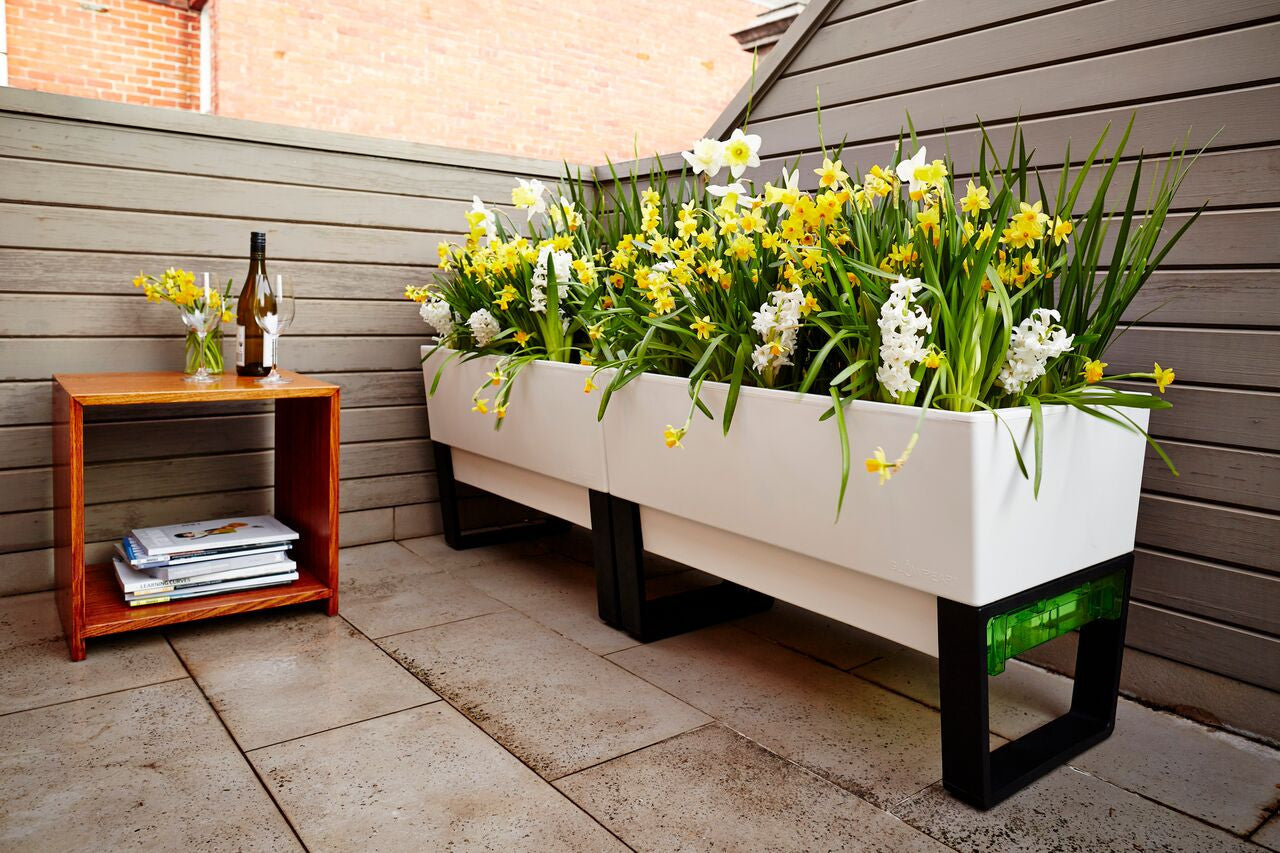This horizontal color photograph depicts a well-maintained patio scene on a sunny day. The focal point is two white planter boxes, each supported by three black legs, which are positioned side by side on a beige tiled floor. The planter boxes brim with vibrant yellow and white flowers, complemented by tall green leaves that create a lush, vertical effect. Adjacent to the planters, on the left-hand side, stands a brown wooden table or shelf, which carries a vase filled with similar yellow and white flowers, echoing those in the planter boxes. The table also holds two wine glasses and a wine bottle, with a few books neatly arranged on a lower shelf. The patio's boundary is marked by a new-looking dark grayish-tan fence, which adds a modern touch to the environment. In the upper left corner of the image, a strip of red bricks decorates the top part of the grayish-tan wall, adding a contrasting rustic element to the setting.